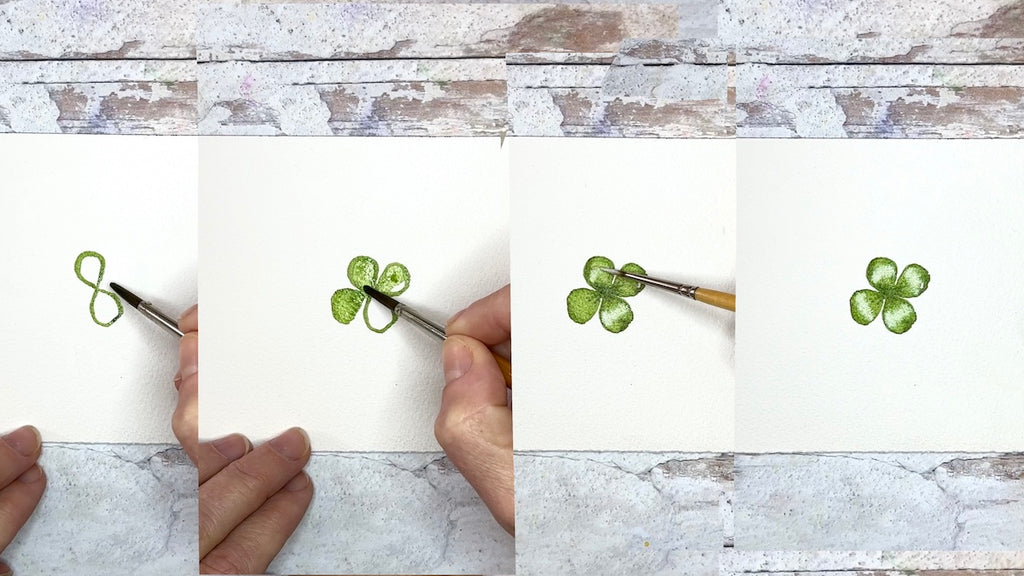This series of four photographs captures the step-by-step process of someone skillfully drawing and painting a four-leaf clover. Each picture is set against a background of a weathered wooden surface that has been painted white and covered with plaster, which is now peeling to reveal the wood underneath. 

In the first photo on the left, the individual begins with drawing a green infinity symbol, resembling the number eight. The tool used, featuring a black tip and a silver handle, is clearly visible along with the artist's fingers. 

In the second image, another green infinity symbol is added diagonally, crossing the first, forming the iconic shape of a four-leaf clover. Three of the leaves are partially colored in, while one remains white.

By the third photo, the artist is seen finishing up with shading, adding white paint to the green leaves to create a reflective shine that gives the clover a more three-dimensional and lively appearance.

The final image showcases the completed four-leaf clover, fully painted with vibrant green and delicate white highlights, set against the vintage-looking, plaster-peeling white wood surface. This sequence offers a detailed and insightful look into the artistic process behind drawing and painting a charming four-leaf clover.